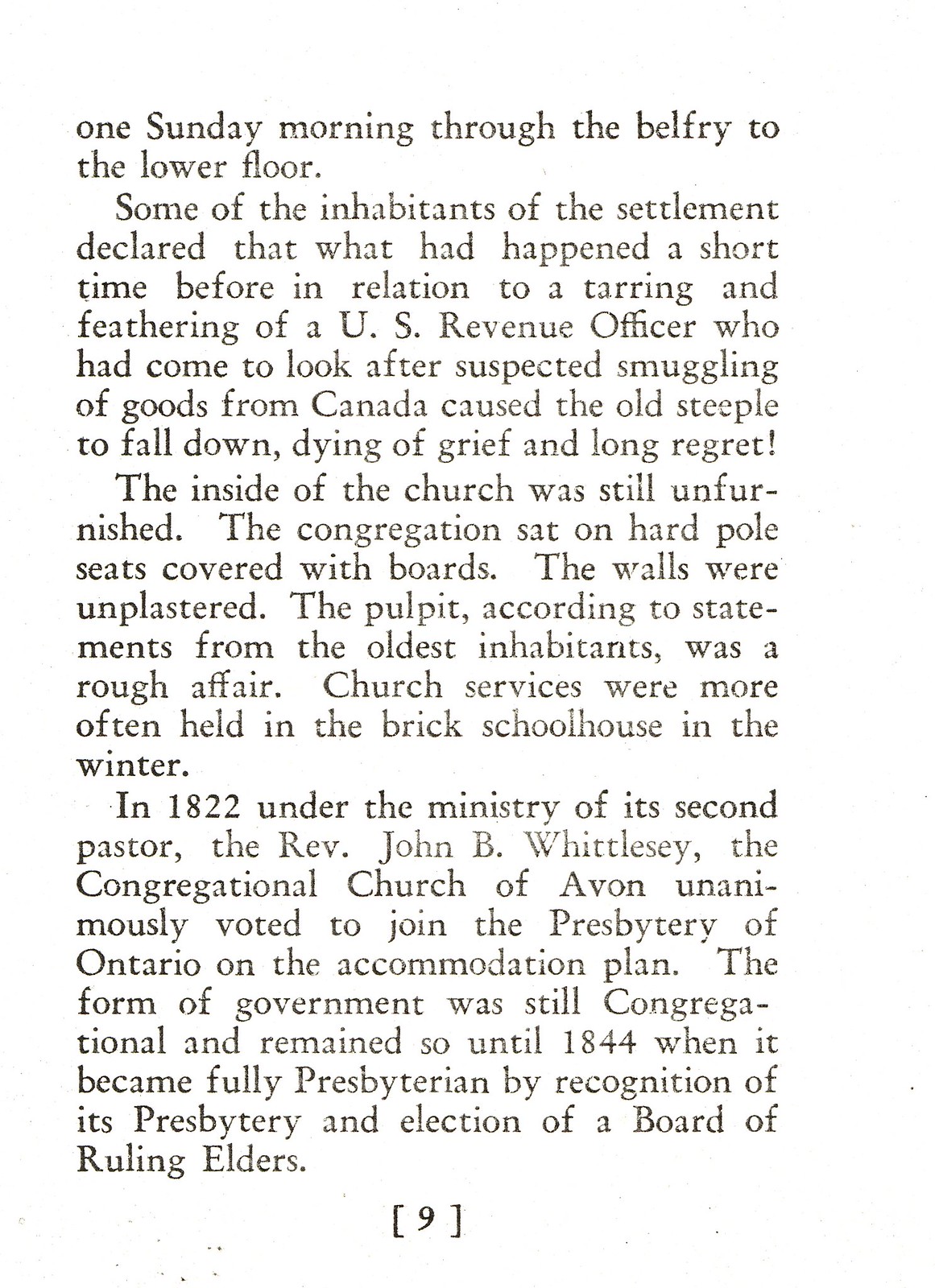The image is of a faded excerpt from a printed book or newspaper, featuring black text on a white background. It details an event that took place on a Sunday morning, where some inhabitants of a settlement believed that the recent tarring and feathering of a U.S. revenue officer—who had been investigating suspected smuggling of goods from Canada—caused the old steeple to collapse, overcome with grief and long regret. At the time, the inside of the church was still unfurnished, with the congregation sitting on hard pole seats covered with boards, and unplastered walls. According to older inhabitants, the pulpit was a rough affair, and church services were typically held in the brick schoolhouse during winter. In 1822, under the ministry of its second pastor, the Reverend John B. Whittlesey, the Congregational Church of Avon voted to join the Presbytery of Ontario on the accommodation plan. The church's form of government remained congregational until 1844, when it transitioned fully to Presbyterian governance by recognizing the presbytery and electing a board of ruling elders. At the bottom of the text, the number [9] is printed, possibly indicating page nine of the source document.